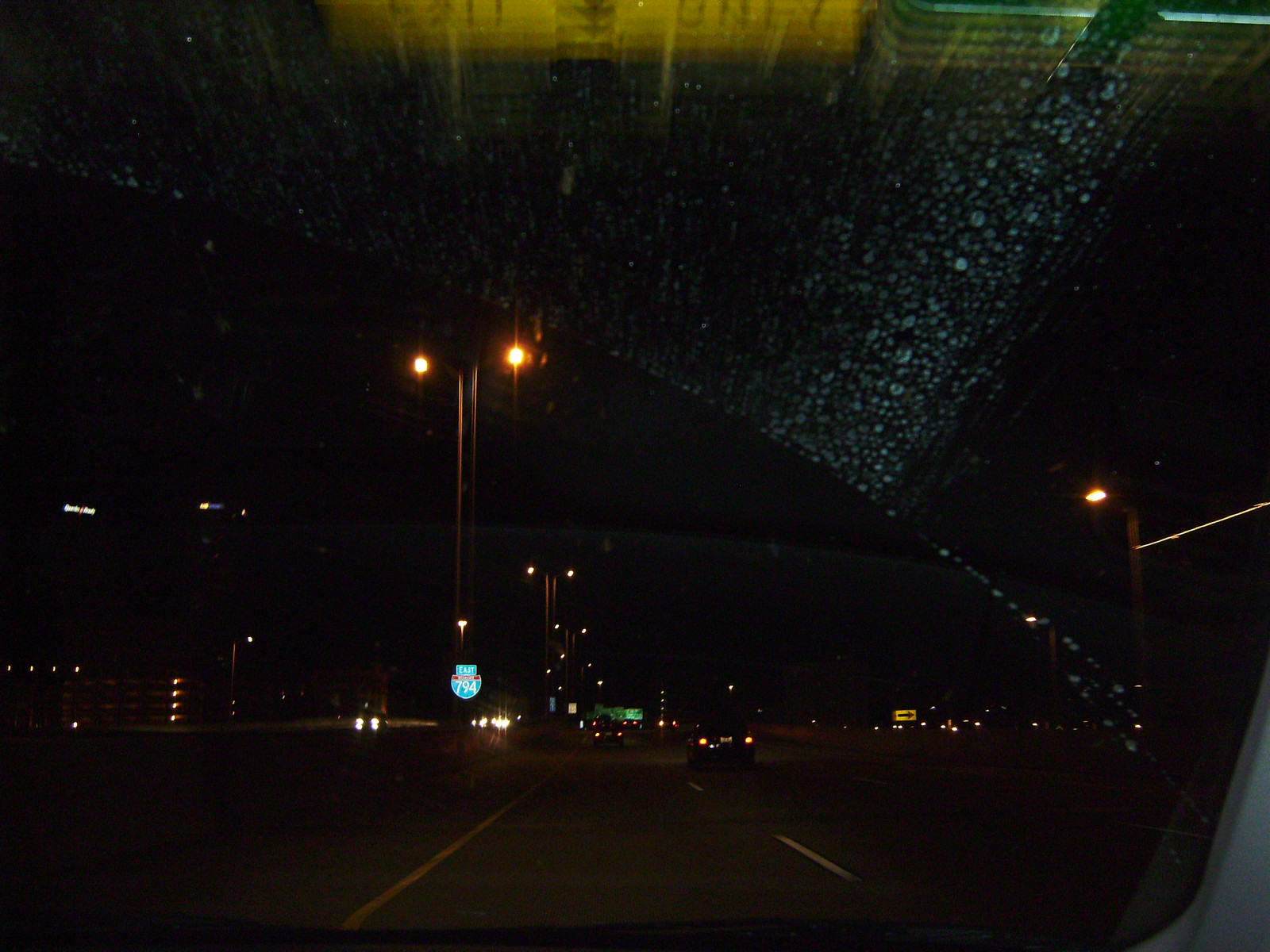The photograph is a nighttime shot taken from the passenger side of a vehicle, looking out through the windshield. The windshield shows clear wiper marks, with the top half of it stained by fluid sprays. The car is traveling in the far left lane of a multi-lane road or freeway. Visible in the scene is a blue highway sign that says "East 794," mounted on a light pole to the left. This light pole features lamps facing both directions to illuminate the road. The photo also shows lane lines, streaks of headlights from oncoming traffic, and a concrete barrier separating the lanes. In the distance, various lights from buildings and road signs are visible, including a green freeway sign ahead and a yellow sign with a right-pointing arrow to the right. The scene is enveloped in darkness, punctuated by street lamps and car headlights.